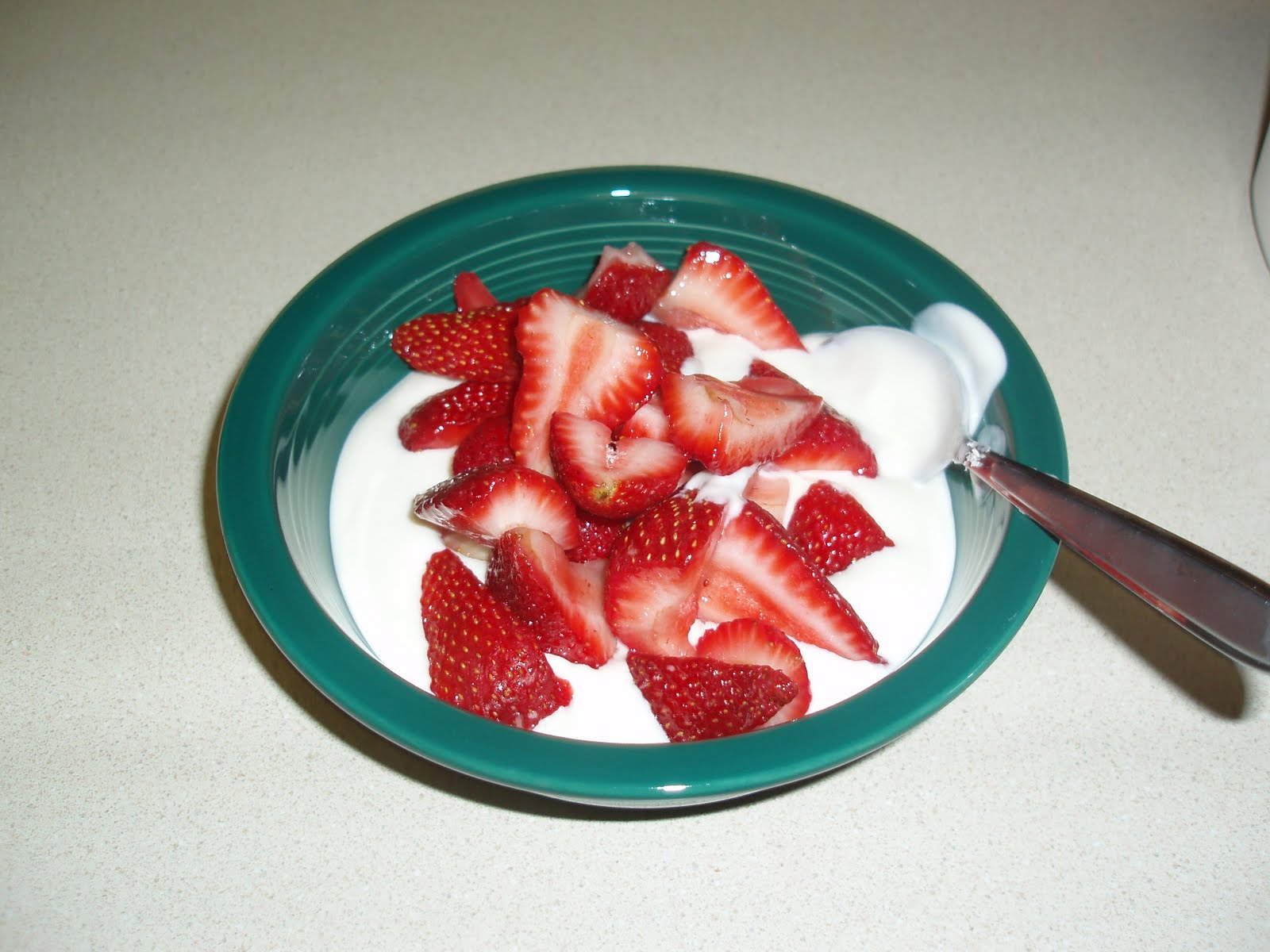A teal-colored bowl sits gracefully in the center of a light, whitish-gray background. Inside, a generous serving of creamy white yogurt forms a pristine base. Atop the yogurt, a mound of juicy, sliced strawberries adds vibrant pops of red, arranged enticingly at the center. To the right of the bowl, a sleek silver spoon awaits, poised for the first delicious scoop. The serene and minimalistic setting enhances the fresh and inviting appeal of this delightful scene.